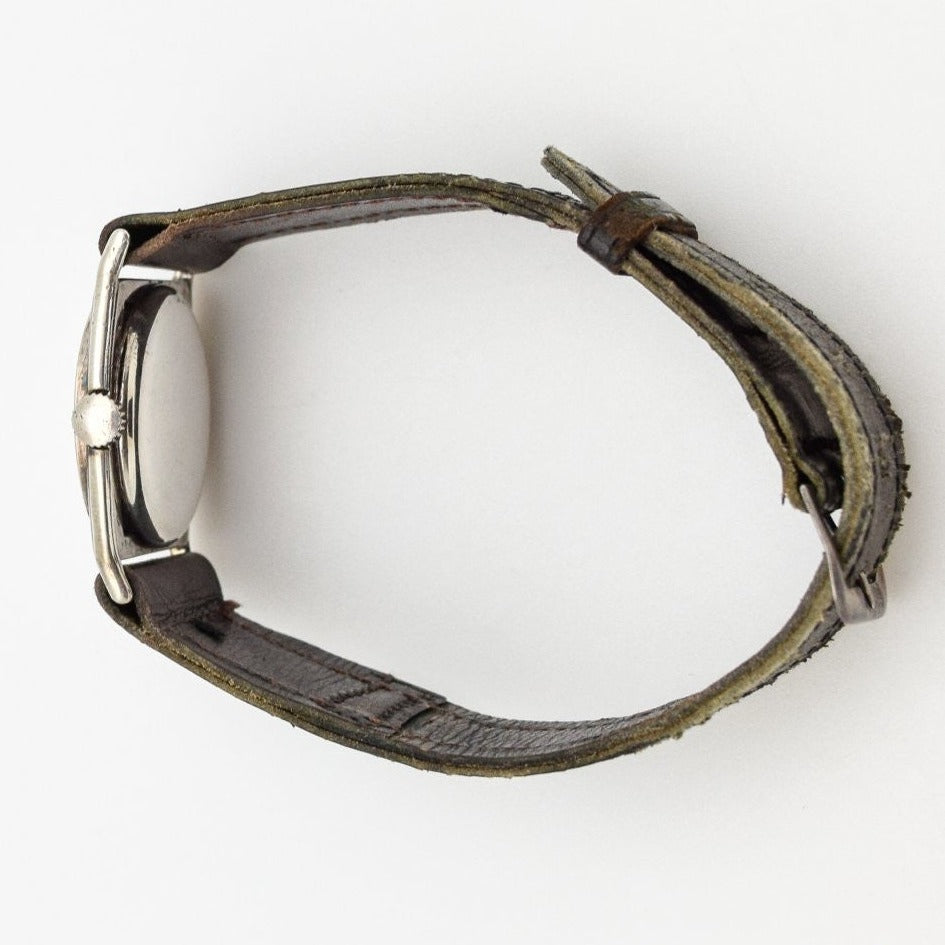The photograph depicts a wristwatch laying on its side against a white or cream-colored background. The watch features a silver, chrome-finished dial with two thin, cylindrical tubes running vertically through the watch strap. The dial, reflecting some light, faces the left side of the image but the watch’s face itself is not visible. Instead, only the polished back of the watch and its adjustment dial can be seen. The watch strap, forming a circle to the right of the watch, is made from worn, rough-textured brown leather with visible stitching on the inside, indicating signs of use. The strap includes a clasp designed like a belt buckle, also in a faded silver color, which appears slightly dog-eared.